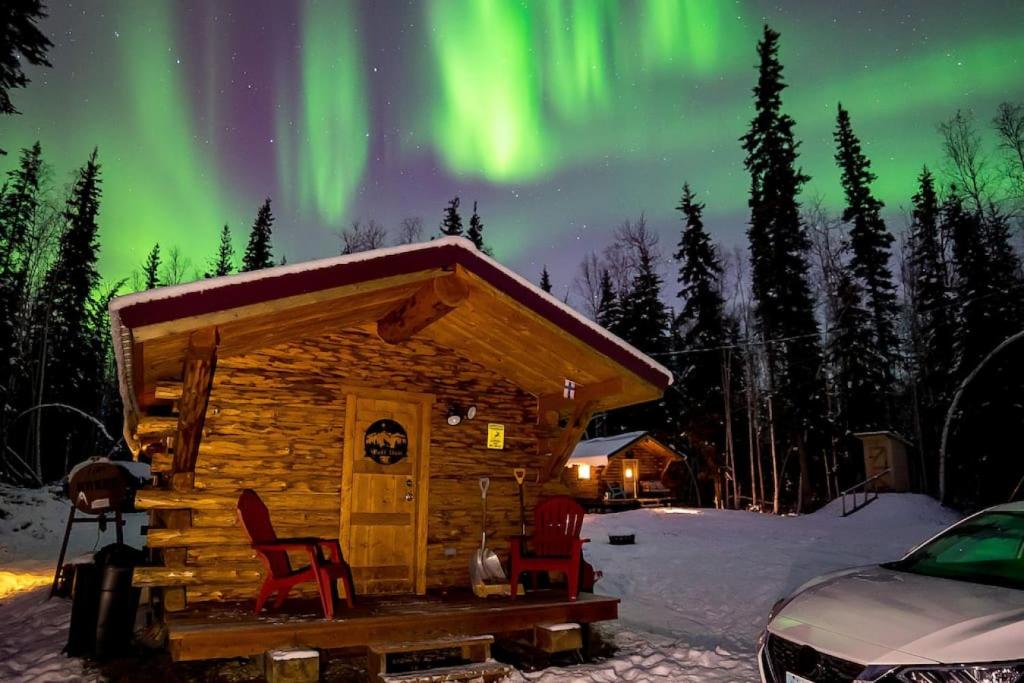In this photograph, the absolutely fantastic image quality captures a stunning winter scene. In the foreground to one side, there is a white vehicle. Opposite it, towards the other side of the image, stands a small wooden cabin constructed from rich, orangey-toned wood. The wood's grain is highlighted with knots and darker streaks. An orangey-colored wooden door complements the two red chairs resting on the porch, signaling a cozy, welcoming vibe. Nearby, a silver snow shovel and an orangey snow shovel are propped up, ready for use. A yellow sign adorns the cabin, flanked by black outdoor lights. Trash cans are visible, adding a touch of everyday realism to the scene.

Above, the sky is nothing short of mesmerizing, with an aurora borealis-like effect showcasing green, white, and lime green hues swirling amongst the stars. Darker patches and vibrant celestial lights intermingle, creating a breathtaking natural display. Snow blankets the ground, accentuating the wintry atmosphere. In the distance, another cabin can be seen, framed by tall, skinny trees that stretch toward the captivating sky. The overall composition renders a picturesque and serene winter landscape, enriched with intricate details and a truly magnificent sky view.